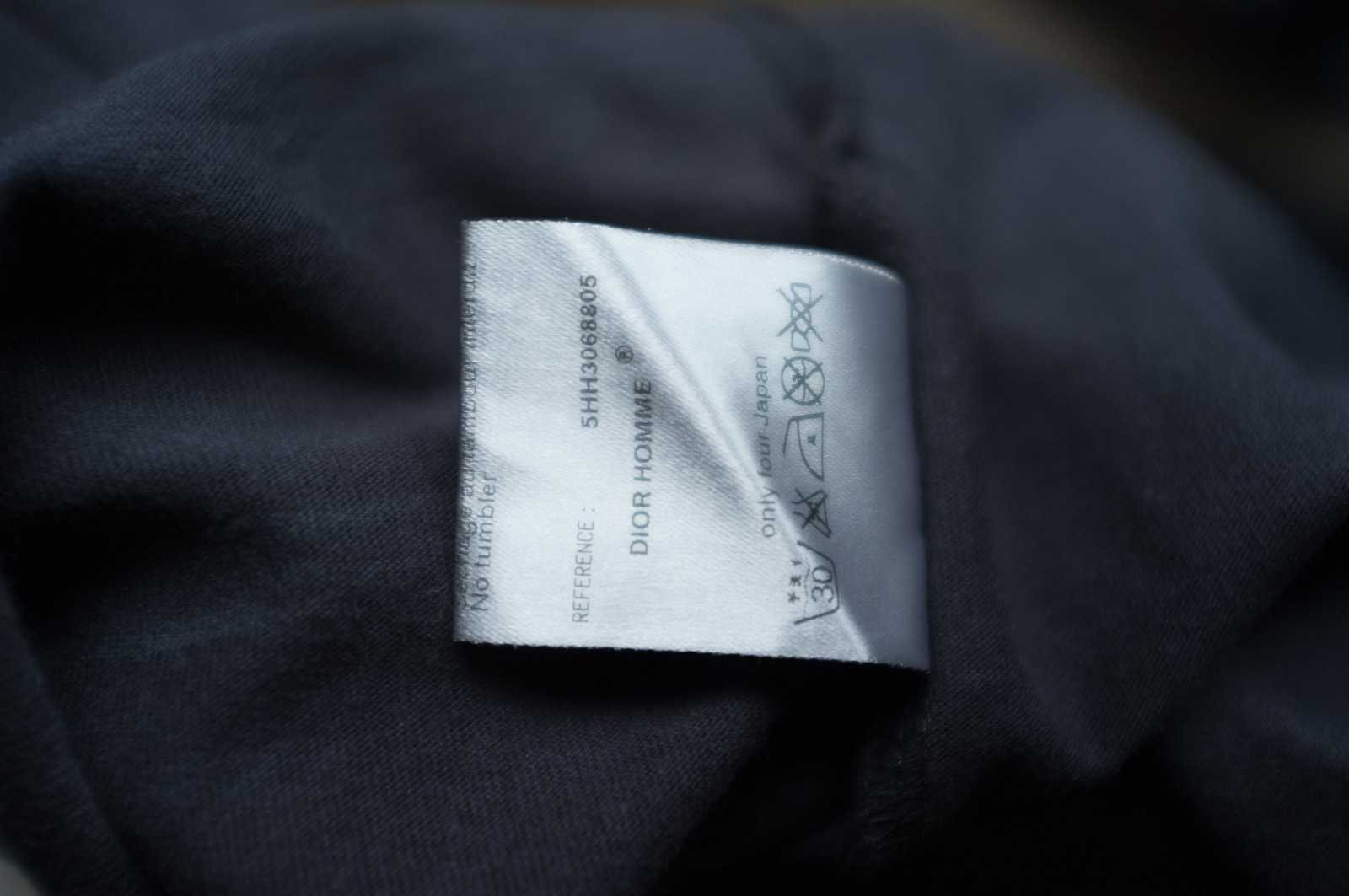This is a close-up color photograph of a garment label stitched into a piece of dark navy or black fabric, though the image is cropped so closely that the exact item of clothing is not discernible. The label, made of shiny satin-like material, appears white with gray shading on its shadowed portions. It is a loop tag sewn into a seam on its right side, leaving the left side free. The text on the label is oriented sideways, requiring a 90-degree anti-clockwise rotation to read it correctly.

Prominently, the label displays the brand name "Dior HOMME" in black font, with a registered trademark symbol (an "R" in a circle) placed to the top right of the "E" in "HOMME." At the top left corner of the tag, the word "Reference" is printed, with a serial number "5HH3068805" on the right side.

Below the brand name, washing instructions include several icons. The first icon, a black bucket with a "30" and three stars above it, indicates a 30-degree washing temperature. The next icon, a conical beaker crossed out, advises against using chemicals. An iron icon with one star indicates ironing at low heat. Two additional crossed-out icons show not to wring the fabric and an unclear symbol, possibly involving a circle with a horizontal line through it.

The text "Only for Japan" suggests a specific geographical usage, although a potential spelling error makes it appear as "Only FOUR Japan." This detailed label not only identifies the garment as part of the Dior HOMME line but also provides essential care instructions, emphasizing restricted use for Japan.